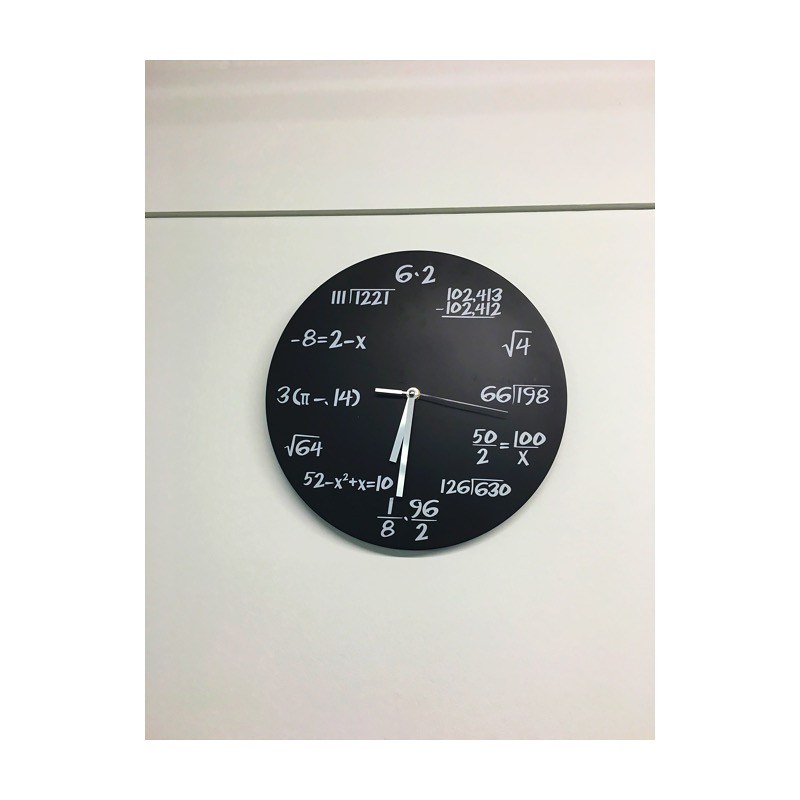The image features an off-white background with a thin, dark gray line running horizontally across it. Mounted on this background is a black circular clock, resembling a vinyl record at first glance. The clock, however, serves as a mathematical joke, as it replaces traditional hour numerals with various mathematical expressions. 

At the 12 o'clock position, the clock displays "6.2." Moving clockwise, other notable positions include the square root of 4 at 2 o'clock, "198 divided by 66" at 3 o'clock, "50 over 2 equals 100 over x" at 4 o'clock, and the square root of 64 at 8 o'clock. The 6 o'clock position features "1.96 over 2." Additional algebraic expressions and fractions replace the rest of the numerals, making the clock an intricate puzzle for the mathematically inclined. All three hands of the clock—hour, minute, and second—are pointing downwards.